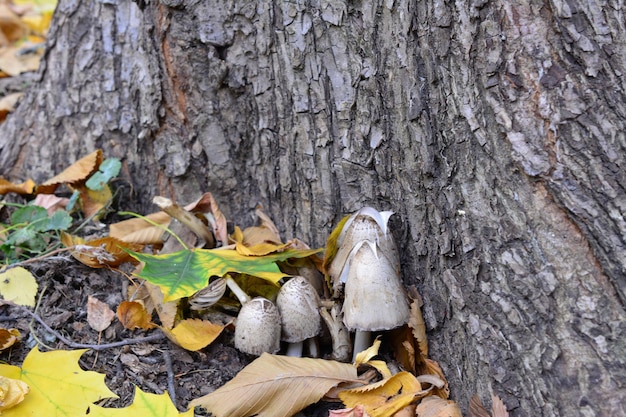This outdoor photograph, likely taken in the fall, captures the base of a thick, rugged tree trunk that possibly resembles an oak. The ground around the tree is littered with an assortment of leaves displaying autumnal hues—yellows, oranges, and browns—many of which are curling up, indicating the season. Among the leaves, several twigs are scattered, and a small patch of ground soil is visible through an opening in the foliage. The main focal point is a cluster of four to five mushrooms with tall stems and elongated, greyish-white caps growing at the tree's base. The lighting suggests an overcast day, enhancing the subdued, earthy tones of the scene.